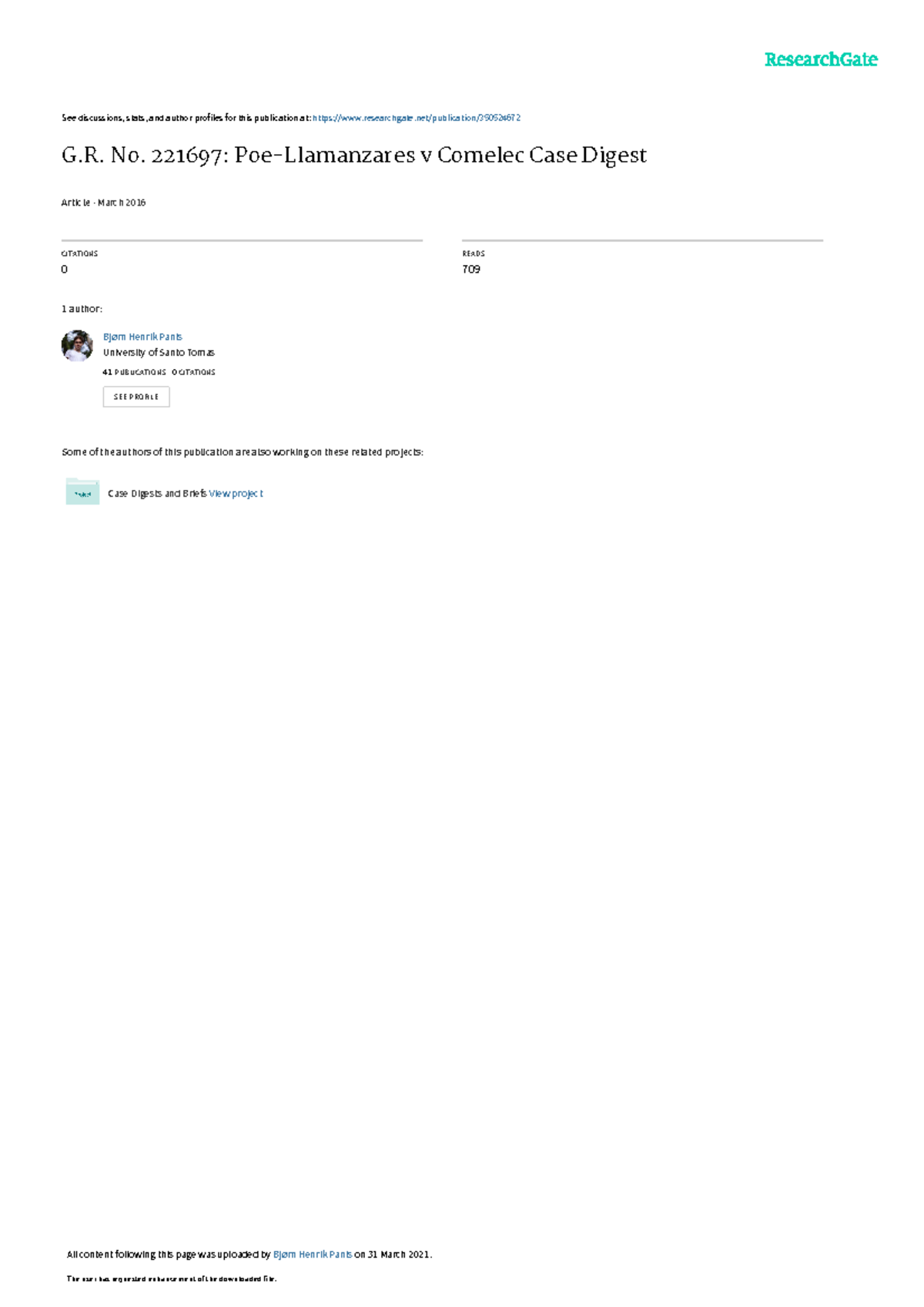This image depicts a largely blank white page with minimal, yet detailed content primarily focused on a publication displayed through ResearchGate. The top right corner bears the green ResearchGate logo. Dominating the middle section of the page, in the largest text size, is the reference number and title: "G.R. Number 221697: Poe-Llamanzares v. Koumelec Case Digest," marked as an "Article" dated March 2016. Below this title, two horizontal lines appear with specific figures: one annotated with "zero" on the left and "709" on the right.

A blue hyperlink, suggesting it leads to ResearchGate.net, invites readers to view discussions, statistics, and author profiles related to the publication. The page features a small author section showing a profile picture, and a partially legible author's name, possibly "Paris," affiliated with the University of Santo Tomas. This author has 41 publications and encourages viewers to "See Profile." 

Additionally, there are mentions of related projects under the section title "Case Digests and Briefs," prompting users to "View Project." Fine print text occupies the bottom of the page, although it remains indistinct in this description.